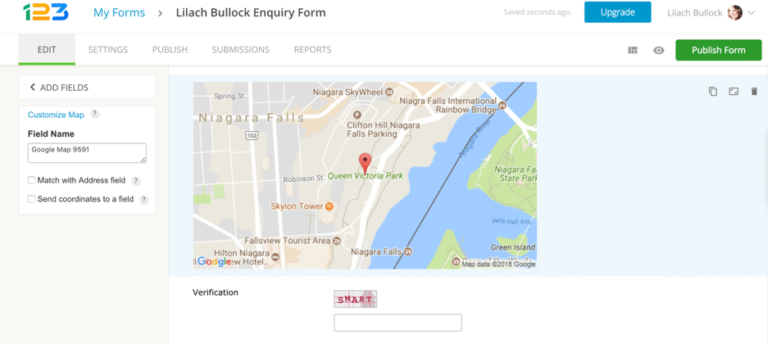In the upper left corner of the image, there are three numbers: 1, 2, and 3. The number 1 is in green, the number 2 is in orange, and the number 3 is in blue. To the right of these numbers, the text "My Forms" is displayed in blue. An arrow pointing to the right directs attention to the text "LILACH BULLOCK Inquiry Form," with each word clearly spelled out and verified as "LILACH BULLOCK" (B-U-L-L-O-C-K). 

Further to the right, there is a blue square with the option to click on it, labeled "Upgrade." Below this, the name "LILACH BULLOCK" is reiterated alongside a circular icon containing an image of a woman with brown hair.

Underneath, there are several actionable options such as "Edit" (underlined in green), "Settings," "Publish," "Submissions," and "Reports." Positioned to the far right, inside a green rectangle, is a button labeled "Publish Form."

The bottom section of the image displays a Google Maps area highlighting various landmarks including Niagara Falls, Niagara SkyWheel, Clifton Hill, Niagara Falls Parking, and Queen Victoria Park. Above this, a red circle with a black dot indicates a specific location, possibly the current location of the individual or the point of interest.